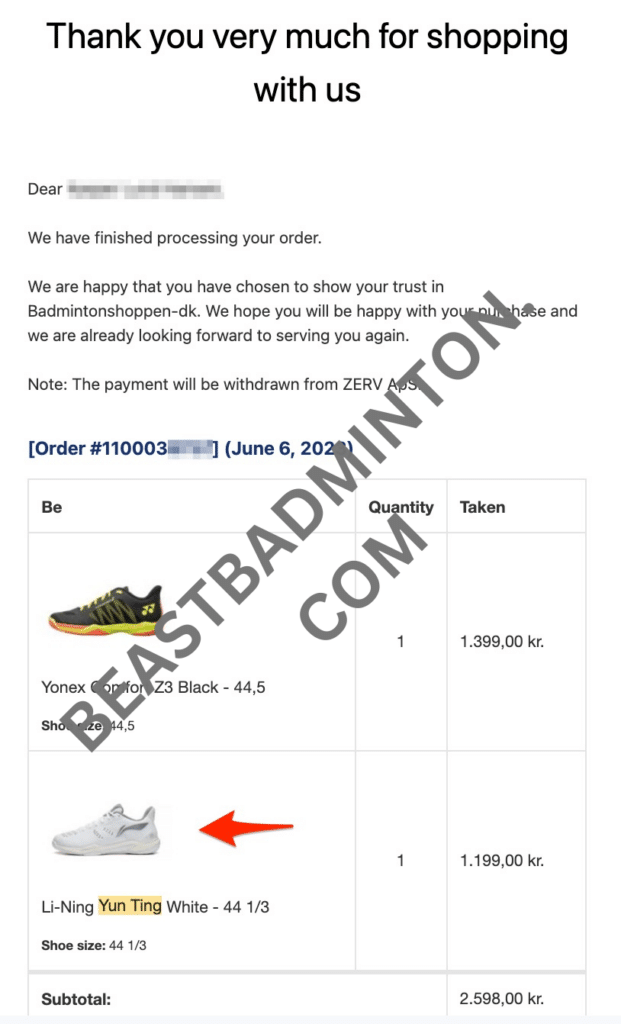**Screenshot of an Order Summary from BadmintonShopping-DK**

The image captures an official thank you letter and order summary from BadmintonShopping-DK. The heading prominently features "Thank you very much for shopping with us." Below this, in smaller type, is a personalized greeting, "Dear [Name]," with the name grayed out for privacy. The letter continues to express gratitude for the customer’s trust and confirms the completion of the order processing. It reassures that the customer will be happy with their purchase and looks forward to future interactions. A note mentions that payment will be withdrawn through Zerve apps.

Details of the order are as follows:

- **Order Number**: 11-0003 (partially blacked out)
- **Date**: June 6th, 2020 (tentative)

A watermark of "beastbadminton.com" is diagonally placed across the document.

**Order Summary**:

1. **Item 1**: 
   - Description: A pair of athletic shoes, black with a yellow sole
   - Quantity: 1
   - Price: 1,399 kroner

2. **Item 2**:
   - Description: Li Ning Yung Ting, white athletic shoe
   - Quantity: 1
   - Price: 1,199 kroner
   - Notable Details: The name "Yung Ting" is highlighted with a yellow background, and a red arrow points to this item. 

Overall, the screenshot is a clear and detailed order confirmation summary, with emphasis on a specific item through highlighting and annotation.